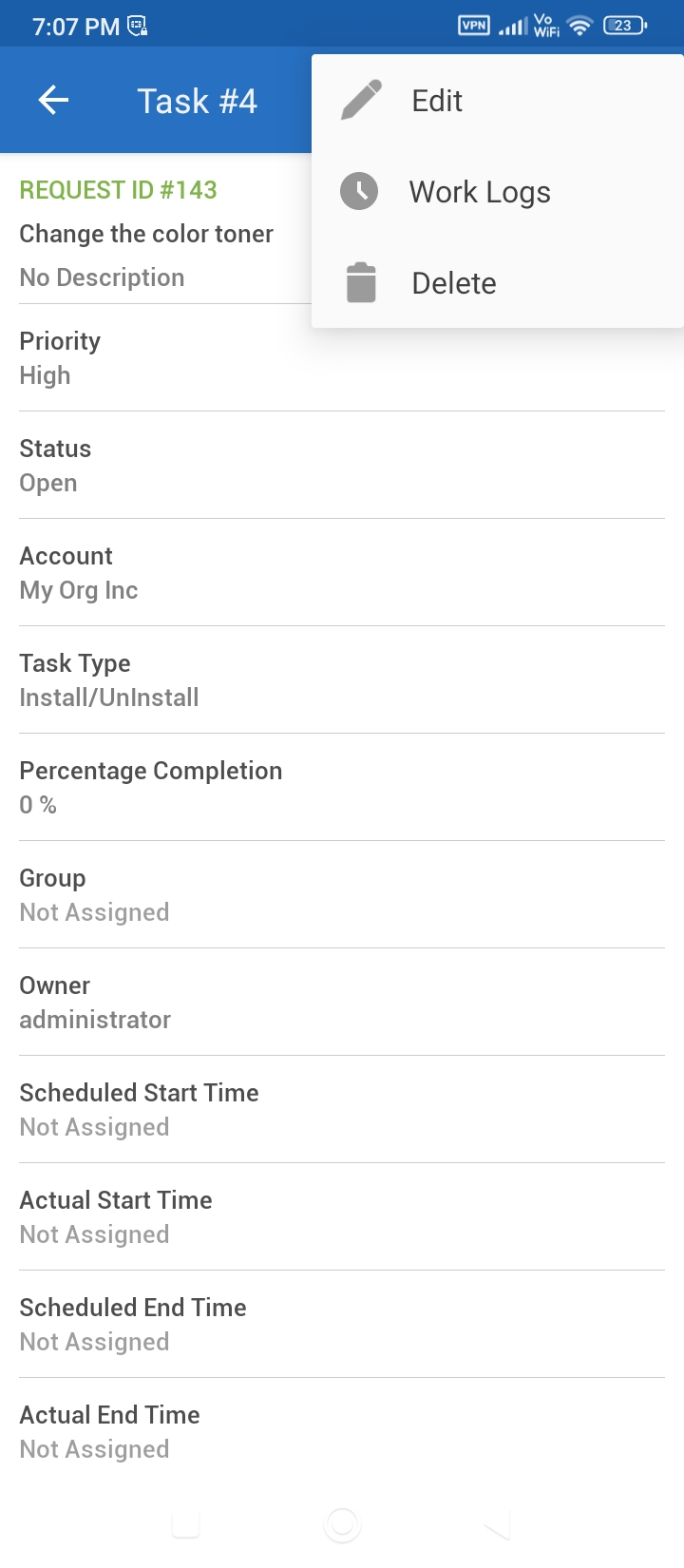A mobile device screenshot showcases a detailed task interface. The device’s status bar indicates it’s 7:07 p.m., connected to a VPN, almost full carrier signal, enabled Wi-Fi, and 23% battery life. The top banner is blue, with an arrow pointing left and labeled "Task Number Four." A pop-up box appears on a lighter blue background, displaying an edit pencil icon, a clock icon labeled "Work Logs," and a delete button with a trash can icon.

Below the banner, the white pop-up features the following details in green text: "Request ID Number 143." Additional information follows in black text, stating the task requires changing the color toner but includes no further description. The priority is set to high, and the status is open. The task is linked to the account “My Org, Inc.,” categorized under the task type "Install/Uninstall." The completion percentage is at 0%, with the group not assigned, the owner listed as "Administrator," and both the scheduled and actual start times not assigned.